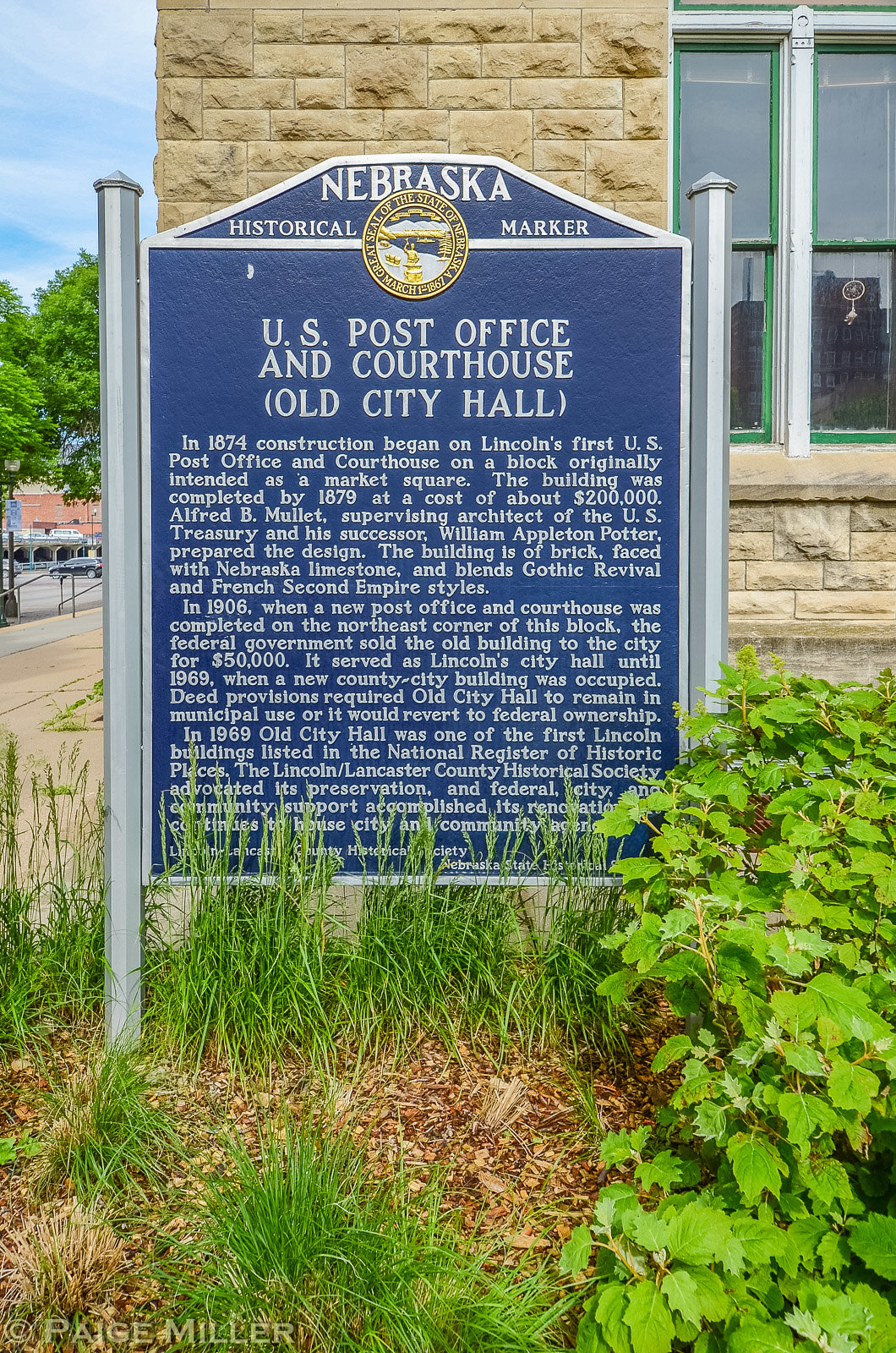This is a vertically aligned rectangular image taken at ground level outside. Dominating the foreground is a tall blue historical marker with silver poles on either side, featuring silver-white text and a gold seal in the center. The top of the marker reads "NEBRASKA HISTORICAL MARKER" in large white caps, followed by "U.S. Post Office and Courthouse, (Old City Hall)" as the title. Below the title, several paragraphs of left-aligned white text recount the building's history. The first paragraph begins with detailing the construction that started in 1874 and provides costs and dates, while subsequent paragraphs outline usage changes over time.

The marker is situated amidst tall grass plants and patches of mulch, with a bush visible on the right-hand side. Behind the marker, there is a brown brick building adorned with windows that have green borders and white trims, typical of a post office. The building suggests it's on a corner, with visible blue skies, white feathery clouds, large green trees in the upper left-hand corner, and windows in the upper right-hand corner. The scene clearly illustrates a historical area in Nebraska during daytime, with distant trees adding depth to the background.